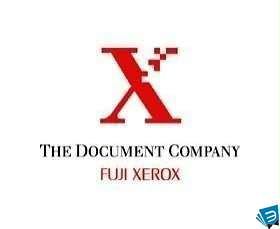This image features a simple yet distinct design centered on a white background, giving it a transparent appearance. Dominating the composition is a capital letter "X" in red, with the top right portion pixelated. The "X" is styled in a font reminiscent of Times New Roman. Below this emblem, in bold black uppercase letters, appears the text "THE DOCUMENT COMPANY," immediately followed by "Fuji Xerox" in red. In the lower right corner of the graphic, there is a small blue element that resembles a fallen book or flag, featuring a white letter that could be interpreted as either a "W" or a backwards "E." This logo is specifically crafted for Fuji Xerox, embodying a modern, minimalistic aesthetic.